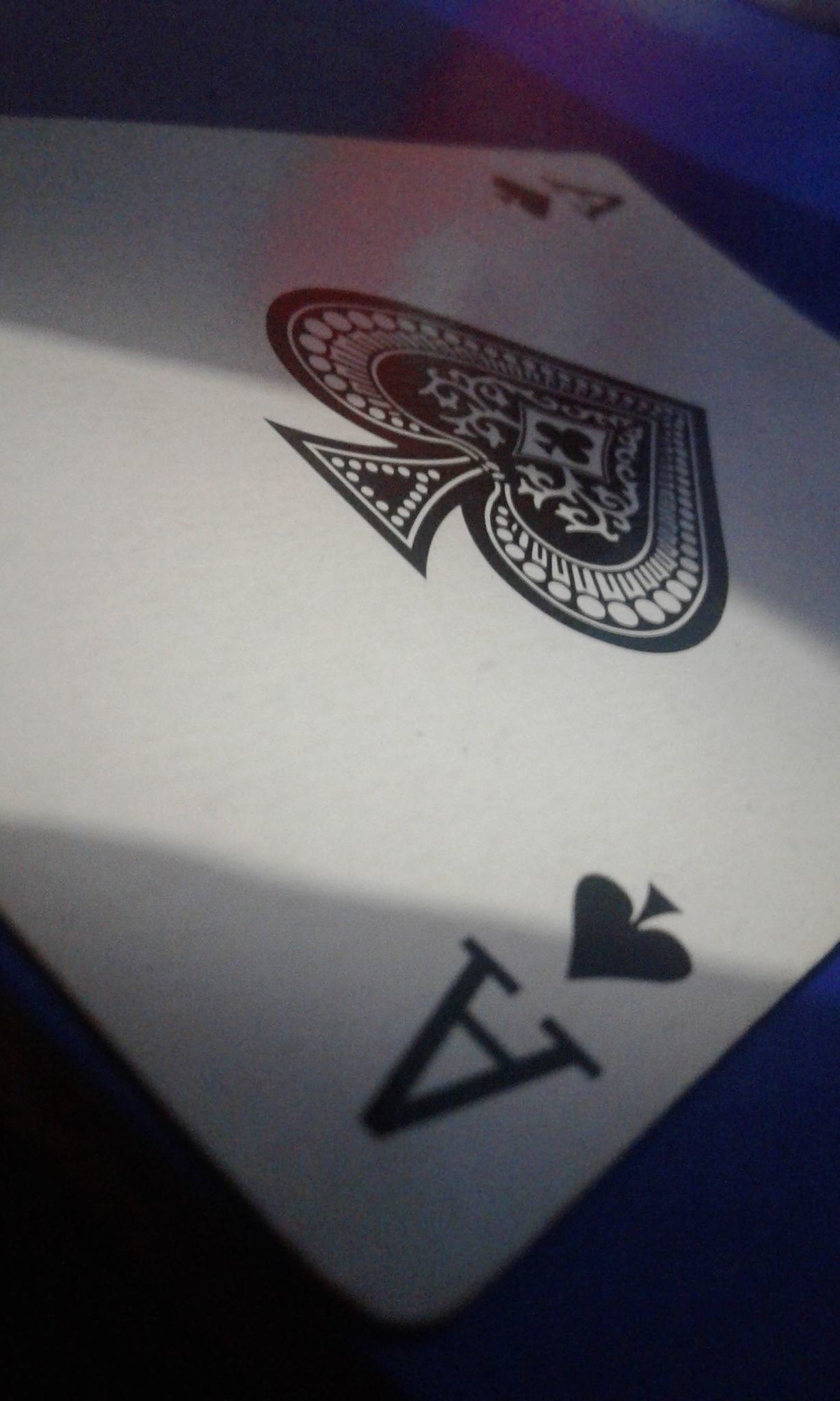This captivating macro photograph showcases an ace of spades playing card in meticulous detail. The image features deliberate focusing, with the front and back parts slightly blurred, while the middle section is sharply defined. The card itself is predominantly obscured by shadows on both the top and bottom thirds, leaving a vibrant, well-lit white band horizontally across the center. 

At the bottom of the card, an upside-down "A" and a spade symbol sit prominently. The centerpiece displays a large, ornate spade adorned with an array of dots around its edges and intricate curlicue patterns within. Interestingly, there is a depiction of a club inside a diamond nestled in the center of the spade, adding an unexpected twist to the design. 

In the top right corner, albeit much more subdued and out of focus, lies another "A" and a smaller spade symbol, partially shrouded in shadow. The lighting effect in the photograph accentuates the middle section, creating a stark contrast with the dimly lit top and bottom thirds. This play of light and shadow brings a dramatic and enigmatic quality to the composition, making the ornate details of the ace of spades stand out magnificently.